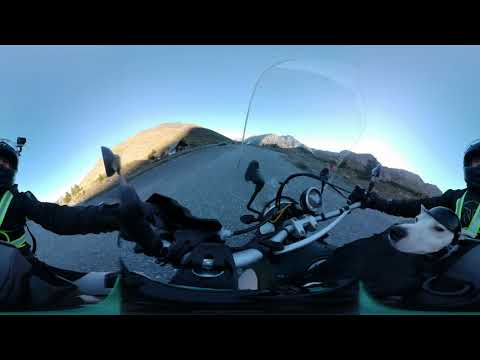The photograph captures a dynamic 360-degree image of a motorcycle ride through a serene countryside, with hills and wide-open roads on either side. At the center of the image, the bike’s green aluminum handlebars and speedometer are prominently visible, complemented by a clear windshield protecting the rider from the wind. The rider, adorned in a black jacket with a neon strip, wears a helmet equipped with a camera on the left side. The unique vantage point of the image offers a slightly warped perspective, depicting the rider on both the left and right sides of the frame. 

In front of the rider, perched on the bike, sits a small white dog adorned with a tiny black helmet, its face clearly visible on the right side of the image. The scene unfolds along a gray roadway winding through rural terrain, flanked by mountain ranges. The left side of the image is bathed in sunlight, illuminating parts of the mountains, while the right side remains in shadow. The sky above transitions from a light blue at the horizon to a deeper blue as it ascends, creating a striking backdrop. The image is bordered by thick black strips at both the top and bottom, adding to its distinct panoramic character.